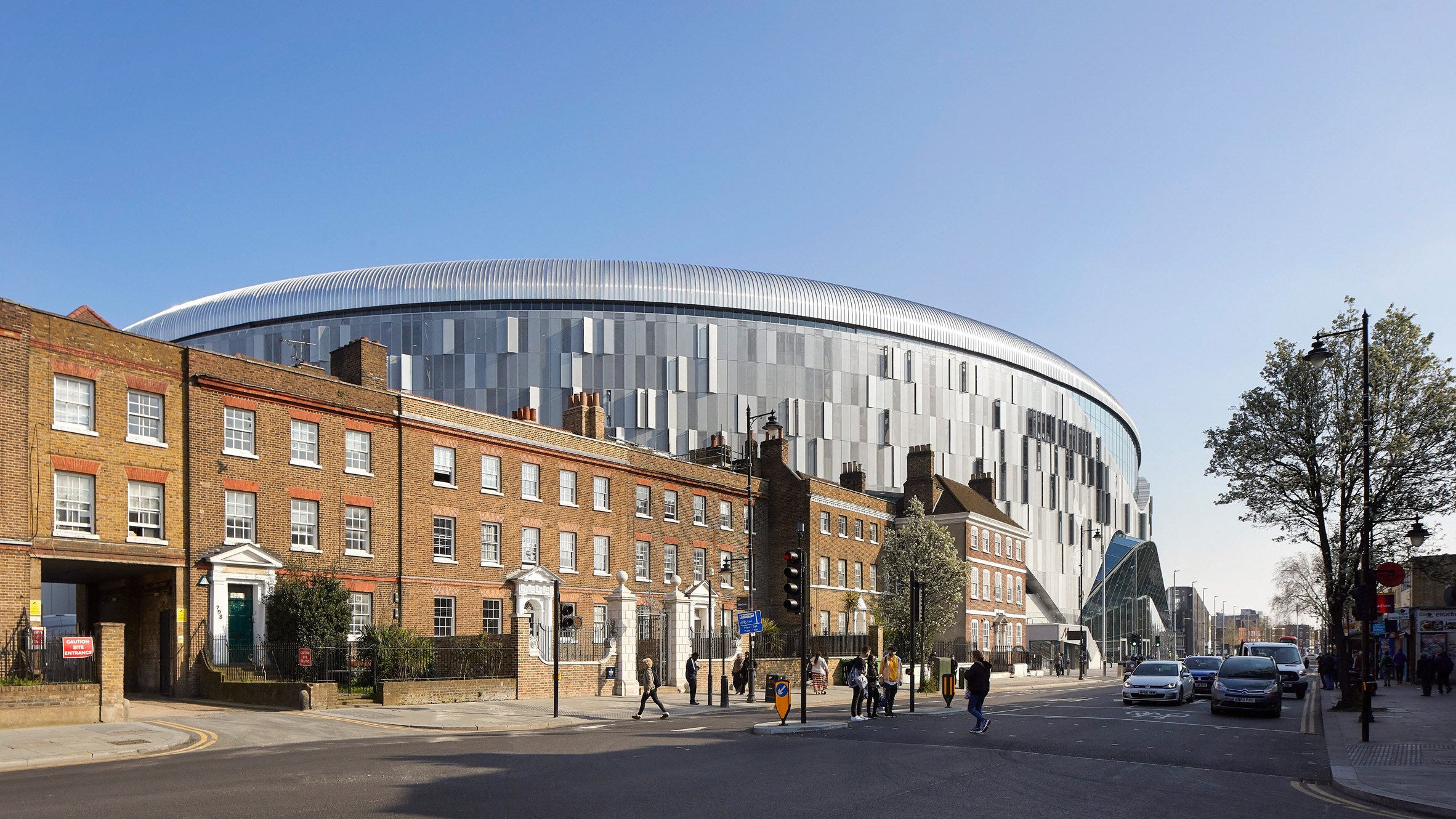The photograph captures a vibrant urban scene under a clear, bright blue sky devoid of any clouds. Dominating the image is a large, circular building adorned with silver, aluminum-like metal panels that gleam in the sunlight. The building, which suggests the form of an amphitheater or stadium, features a distinctive top section accentuated with colorful elements. In front of this striking structure is a brown multi-storied row house that appears to be part of a college campus or residential area. The street before the buildings is busy with both parked and moving cars, and people casually walking in a nonchalant manner, going about their daily routines. To the right side of the image, a tree grows along the sidewalk, providing a touch of greenery to the urban landscape. The harmonious blend of architectural elements and human activity creates a dynamic snapshot of everyday city life.